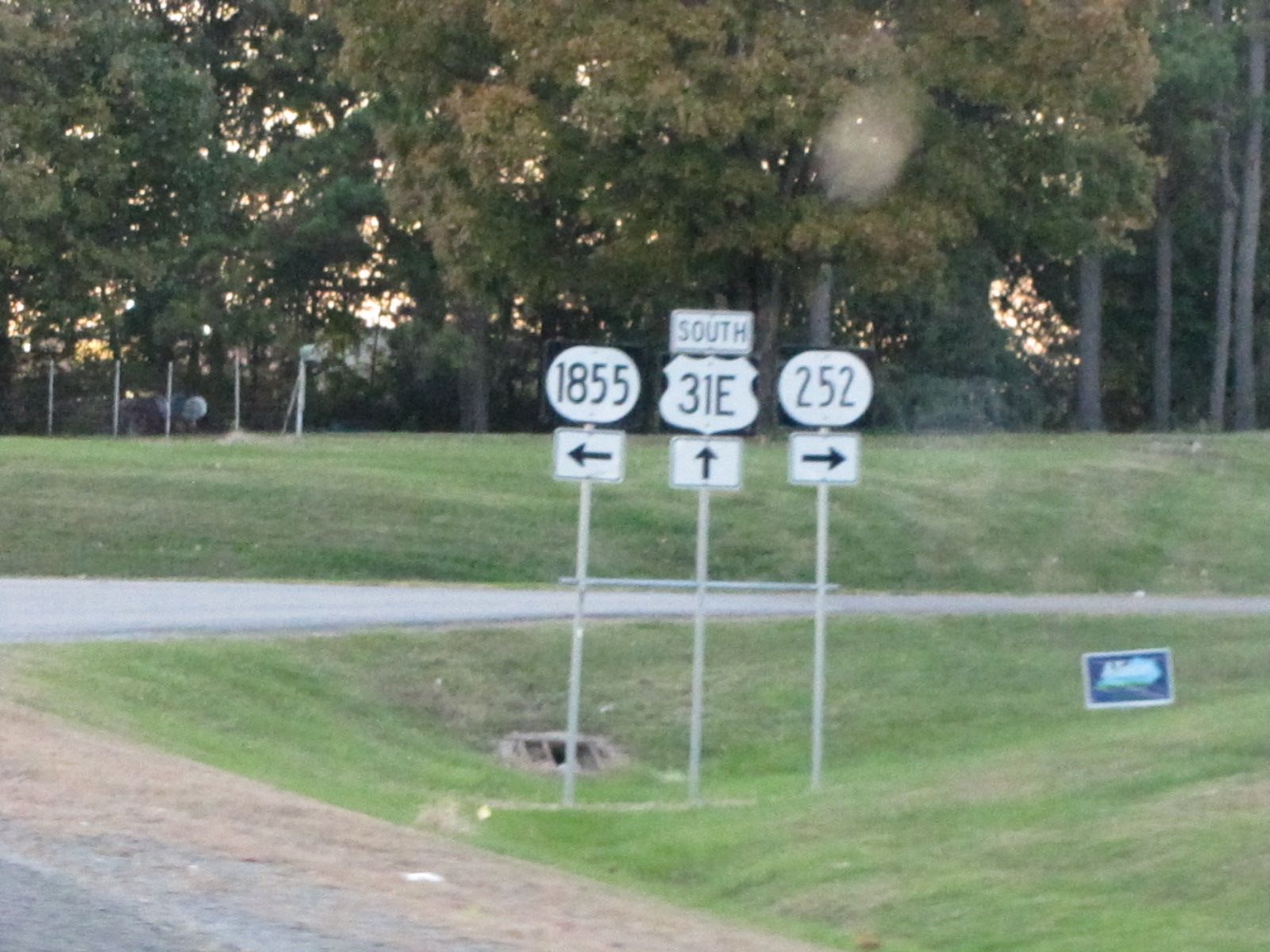This outdoor image, captured during dawn or dusk, showcases a tranquil scene with a thick grouping of green trees in the background, partially illuminated by soft sunlight. The foreground features a gently sloping grassy hill, encircled on the left by a small barbed wire fence. At the base of the hill, a road runs horizontally, bordered by a grassy patch containing a drainage grate. On the left lower corner, another road is visible. Alongside the grassy patch, there is an election sign. Prominently, three black and white directional signs are standing on the green grass: the first sign reads "1855" with an arrow pointing left, the middle sign reads "South 31E" with an arrow pointing up, and the third sign displays "252" with an arrow pointing right.